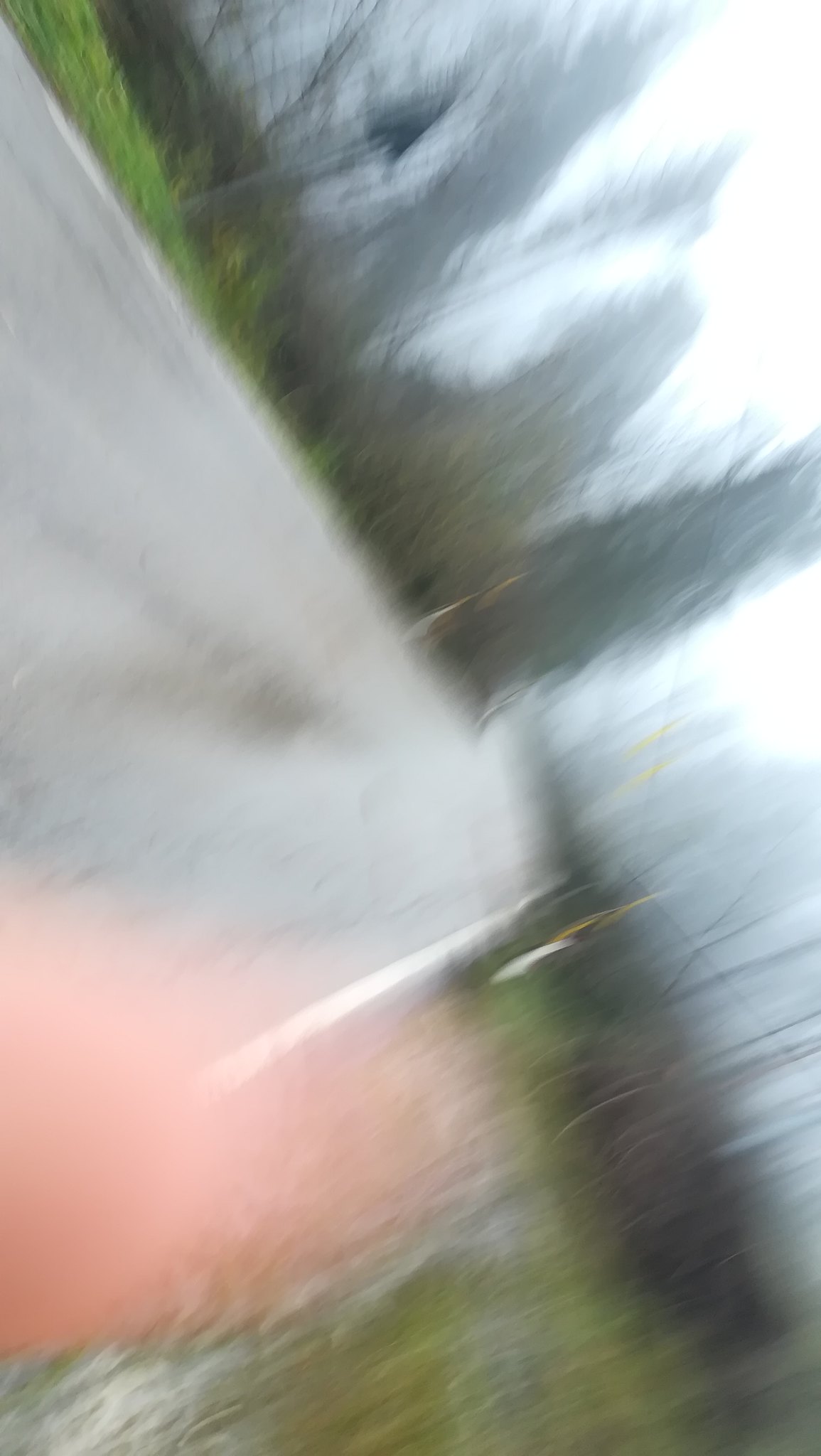This vertical, blurry photograph appears to capture a rural two-lane road, possibly gravel or cement, bordered by dense trees. The majority of the trees are bare, suggesting the photo was taken in fall or winter, interspersed with evergreen pines. On one side, there is a utility pole visible, likely for electricity. A solid white line delineates the edge of the road. Grass can be seen on the right-hand side, and there might be a reflective surface or water nearby, indicated by a distant light or reflection. The bottom left corner of the image is obscured by what seems to be a finger, likely the index finger or thumb of the person taking the photo.